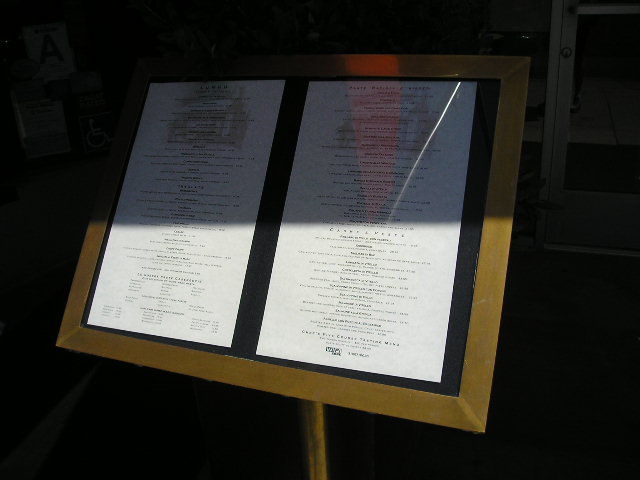This image features a photograph of what appears to be a framed restaurant menu displayed in a stand positioned outside the establishment. The menu is enclosed in a rectangular, golden frame and is oriented vertically. It consists of two pages, although the text on the menu pages is not legible in the photograph. The layout and design suggest it is a high-end or fancy menu, indicated by the sophisticated formatting and the presence of watermark-like images of buildings at the top of each page. 

The lighting in the image creates a contrast, with the upper half of the menu shaded and the bottom half illuminated by sunlight. In the background, a building can be vaguely discerned, partially obscured by shade. This building features architectural elements such as a door or window, adding context to the setting and further suggesting the menu's outdoor placement.